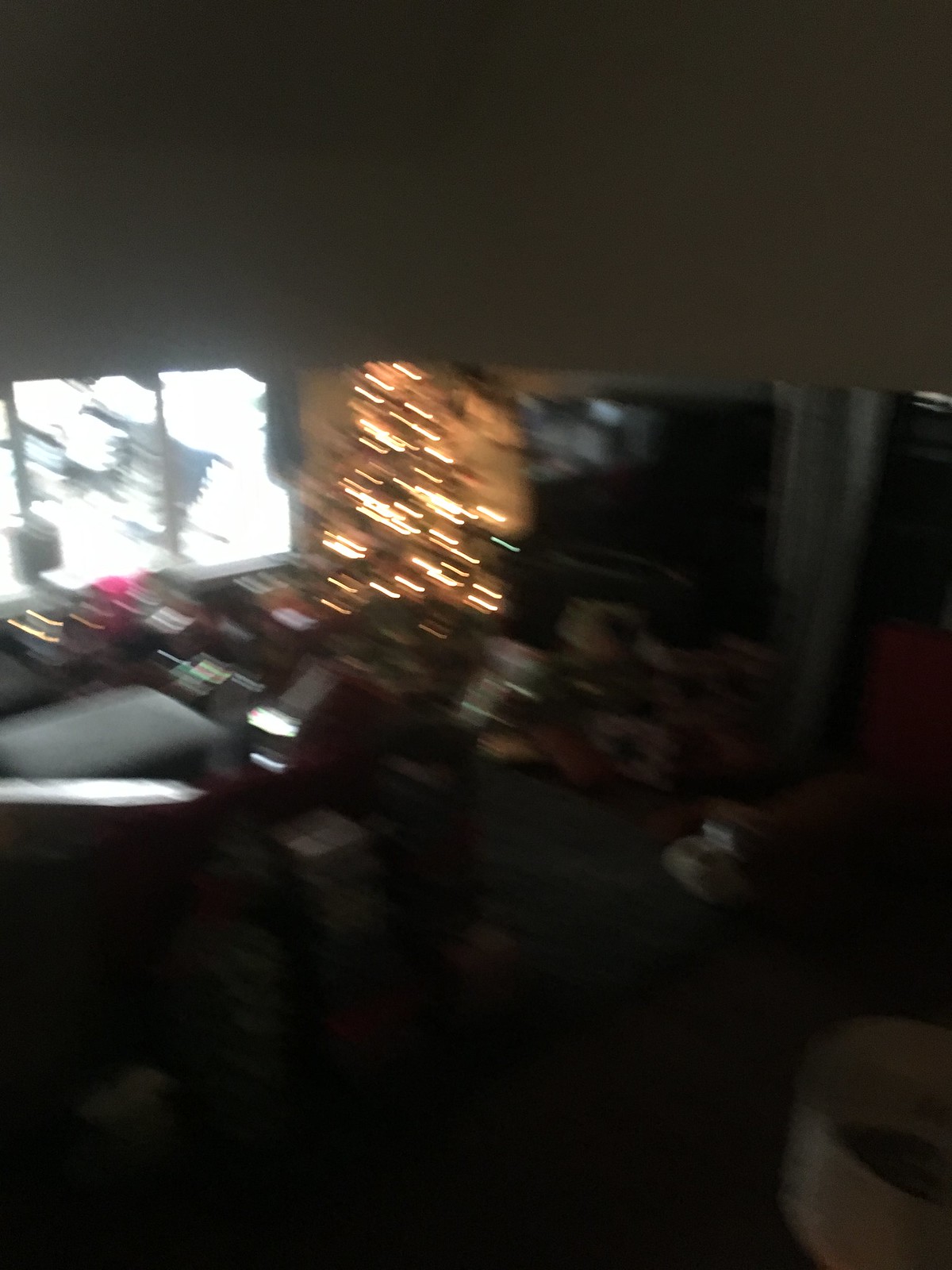This photograph, taken indoors likely in a living room during Christmas time, captures a festive but blurry scene. The focal point is a Christmas tree in the far corner, adorned with bright white lights that illuminate an otherwise dark room. To the left of the tree, there's a window faintly visible. Despite the room's darkness and the image's lack of sharpness, one can discern several wrapped presents scattered around the base of the tree. In the bottom right-hand corner, a flat-screen TV is partially visible behind a white lampshade. A cozy chair with a gray cushion is situated beside the window, adding to the homely ambiance of the room.